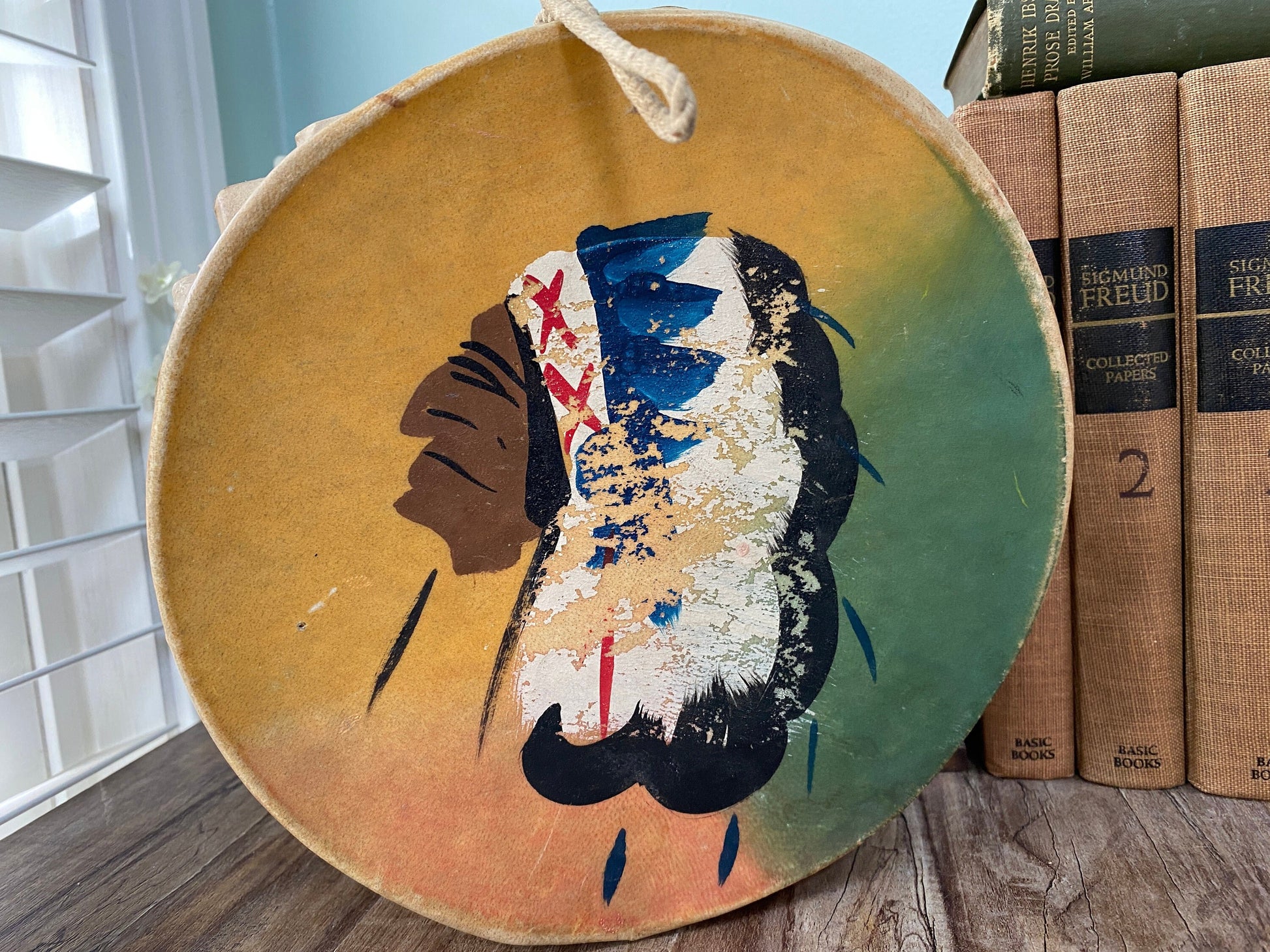In this staged indoor photograph, taken during the daytime with natural light, a wooden table hosts a prominent Native American drum at its center. This circular drum, accentuated by a light cream-colored rope around its edges, features a vibrant portrait of a Native American chief with brown skin, facing left. The chief wears a headdress adorned with white feathers, blue feathers pointing to the right, and red X's, although the paint is peeling off in places, revealing the light cream base beneath. The background of the drum is divided into segments of orange at the top, light green on the right, and light pink at the bottom.

To the right of the drum sits a stack of books, topped by a green box. The books include titles such as "Sigmund Freud: Collected Papers," with the number two visible on one of them. On the left side of the image is a window with white blinds partially opened, allowing light to filter through and cast a soft glow on the scene. The backdrop features a blue or teal-colored wall, adding a subtle contrast to the composition.